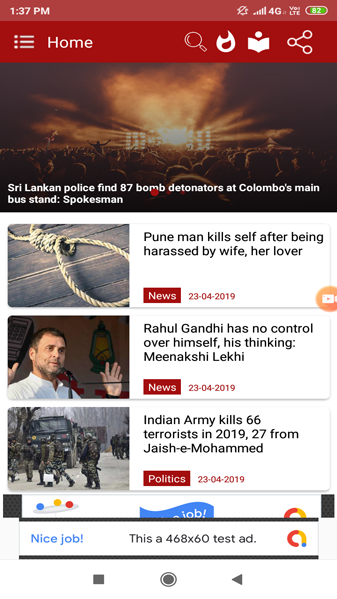This image is a detailed screenshot of a person's mobile phone screen, containing several user interface elements and news headlines. 

At the very top of the image is a red status bar, displaying white text indicating the time as 1:37 p.m. and the phone's battery percentage at 82%.

Below the status bar is a darker red navigation banner that reads "Home," and includes icons for a magnifying glass, a flame, and a book.

The main section of the screenshot showcases a color photo taken at night, featuring a crowd in front of a bright light. Accompanying this image is a news headline stating, "Sri Lankan police find 87 bomb detonators at Colombo's main bus stand: spokesman."

Beneath this, the background transitions to white and displays three separate news stories, each paired with a photo and a headline:

1. The top photo depicts a noose, accompanied by the headline, "Pune man kills self after being harassed by wife, her lover. 23-04-2019."
   
2. The middle photo is a headshot of a man, with the headline reading, "Rahul Gandhi has no control over himself, his thinking: Meenakshi Lekhi. 23-04-2019."
   
3. The bottom photo shows uniformed troops on a road, with the headline, "Indian Army killed 66 terrorists in 2019, 27 from Jaish-e-Mohammed. 23-04-2019."